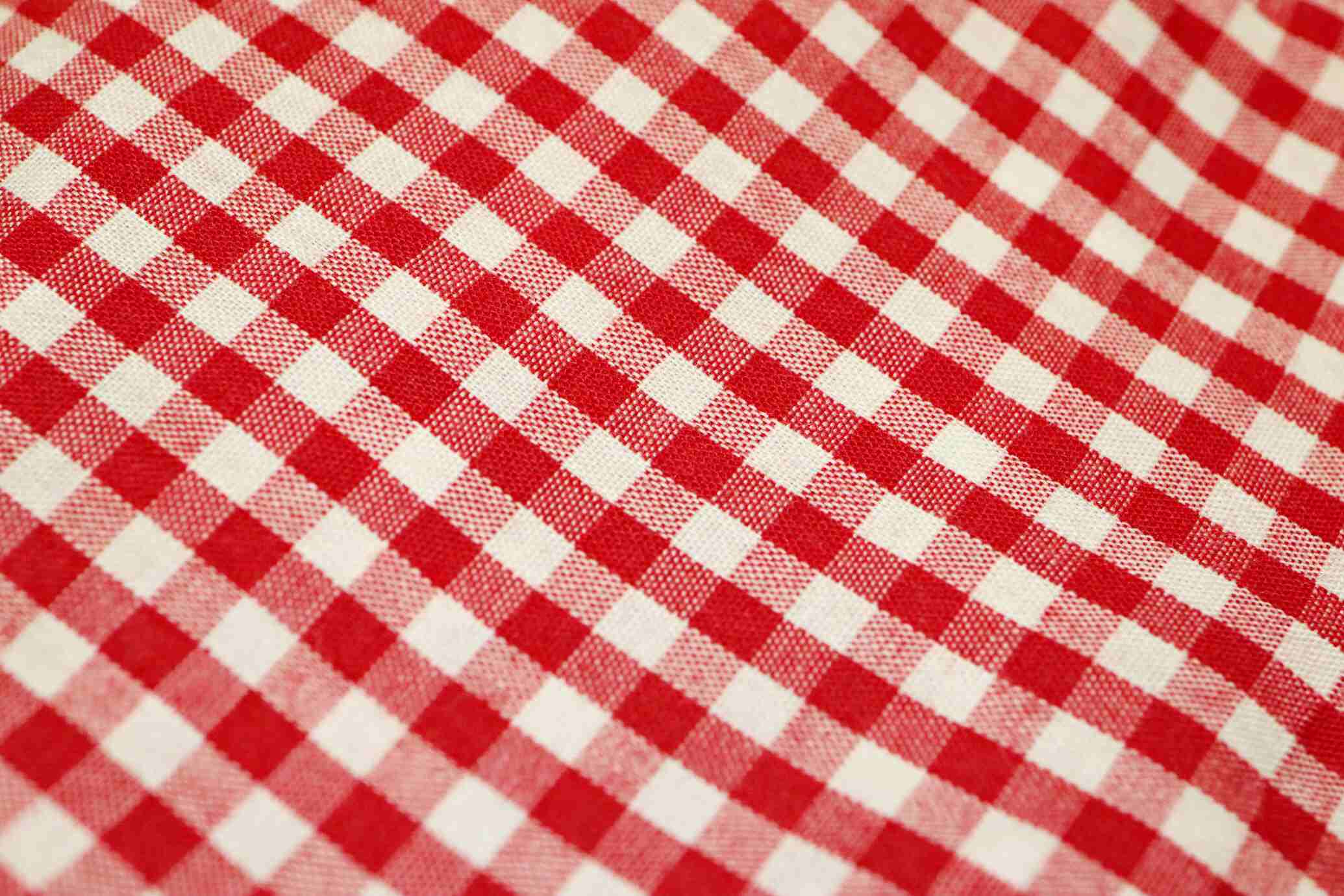The image is a detailed close-up of a red and white plaid fabric, possibly a tablecloth, handkerchief, or shirt. The pattern consists of a symmetrical grid formed by intersecting red and white lines, creating a series of squares. Within these squares, the red and white colors blend and intersect symmetrically, with varying intensities, including darker and lighter shades of red. The cloth appears slightly uneven, notably with a minor sway in the upper right side, disrupting the flow just a bit. The corners, particularly the upper left and bottom right, are out of focus, while the center remains the sharpest. The overall effect is a consistent and repeated pattern, though some areas show more dominance of white or red. The fabric's surface appears to be on an uneven surface, contributing to the slight blurriness observed in the lower portion of the image.